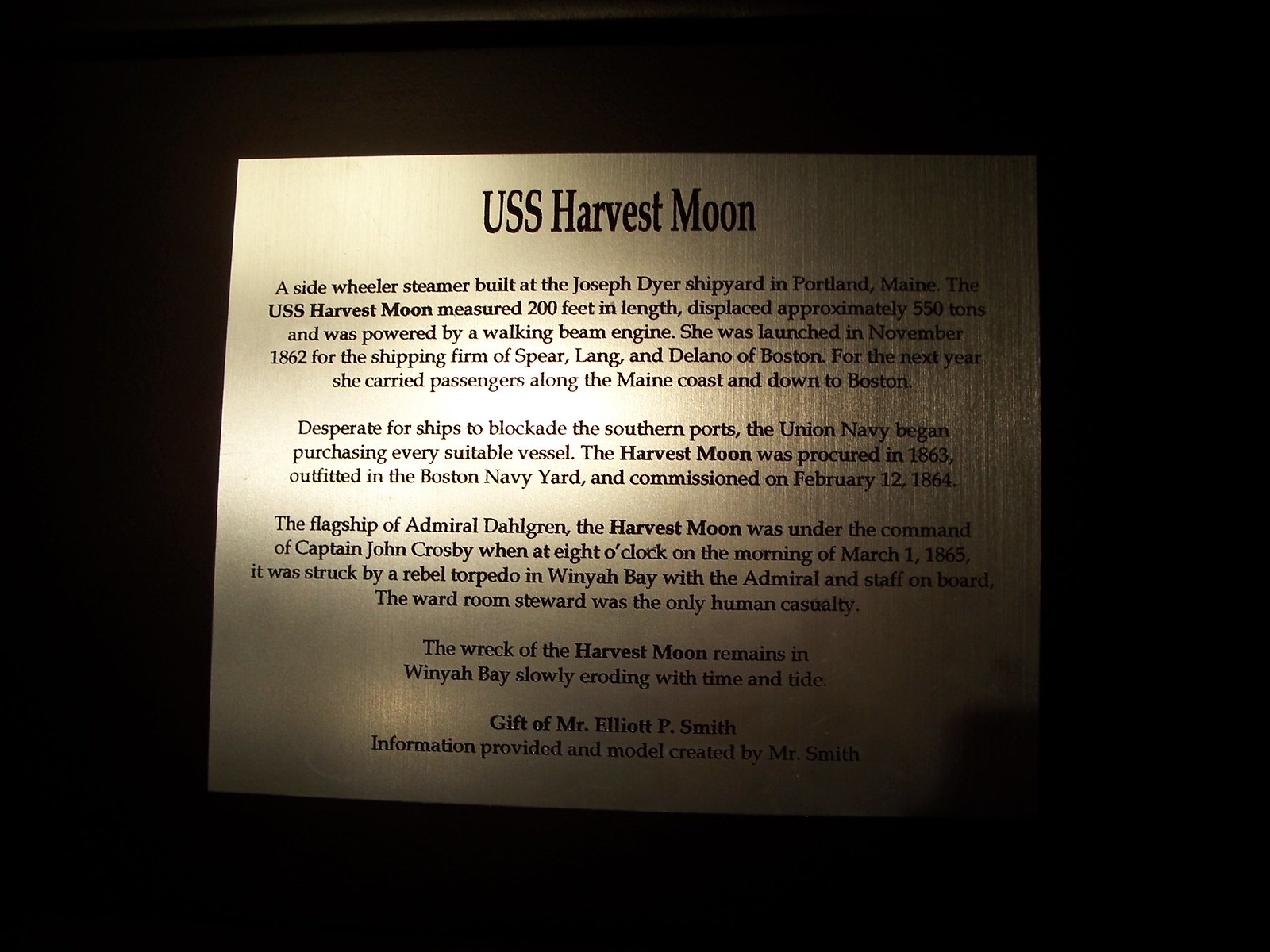Presented in a meticulously recreated museum setting, the display features a black background with dim lighting that highlights a prominent white placard titled "USS Harvest Moon" rendered in black typeface. This descriptive plaque is centered and surrounded by details that provide a thorough historical account of the vessel. 

Built at the Joseph Dyer Shipyard in Portland, Maine, the USS Harvest Moon was a sidewheeler steamer that stretched 200 feet in length and displaced approximately 550 tons. Powered by a walking beam engine, the ship was launched in November 1862 for the shipping firm Spear, Lang, and Delano of Boston. During her initial year, she transported passengers along the Maine coast and down to Boston. 

As the Civil War intensified, the Union Navy, desperate for vessels to blockade Southern ports, acquired the Harvest Moon in 1863. She was outfitted at the Boston Navy Yard and commissioned on February 12, 1864. The ship served as the flagship of Admiral John A. Dahlgren and was under the command of Captain John Crosby. 

Tragically, on the morning of March 1, 1865, the Harvest Moon struck a rebel torpedo in Windham Bay while carrying the admiral and his staff. The wardroom steward was the only human casualty of the blast. Today, the wreckage of the Harvest Moon remains in Windham Bay, gradually succumbing to the ravages of time. 

The display also highlights that this detailed model of the USS Harvest Moon was generously donated by Mr. Elliot P. Smith, who meticulously crafted the replica.